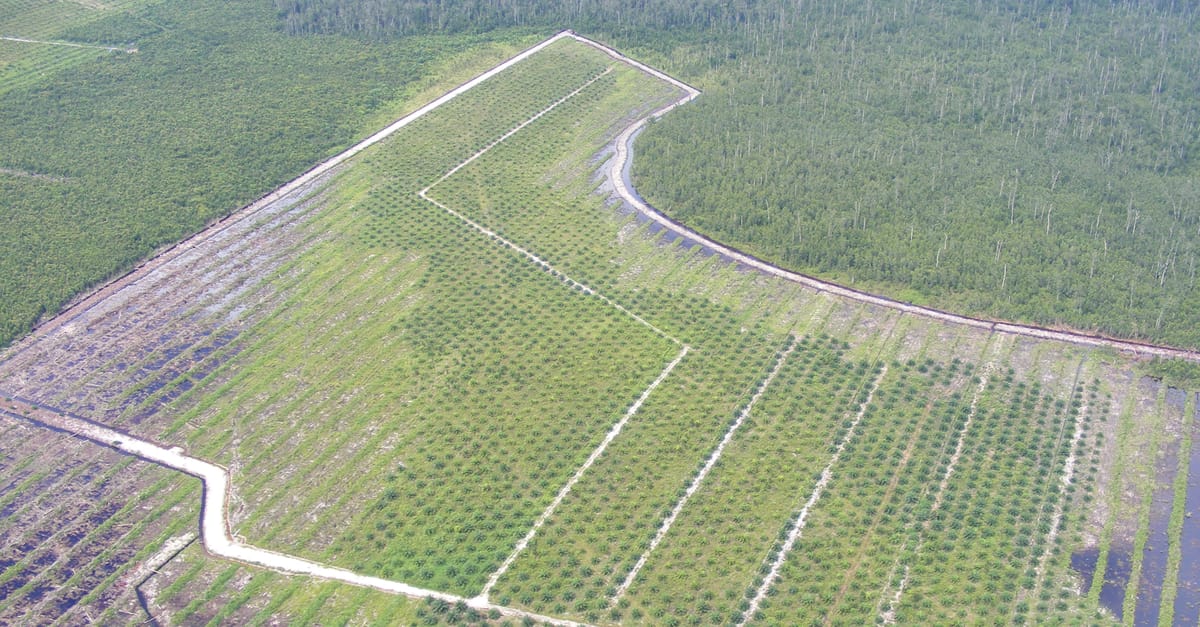This is a horizontally aligned rectangular aerial photograph of a mixed landscape featuring cropland and forest. The top section of the image displays a green expanse of forest, visible both to the left and right sides. In the upper left corner, there is some farmland, identifiable by its alternating light green and dark green stripes. The primary focus of the photograph is the centrally located piece of land, characterized by a white border which likely represents roads or dirt pathways. These white pathways crisscross horizontally and diagonally, indicating infrastructure amidst the land. The lower right section of the image shows these diagonal lines extending to about the middle of the photograph. In the lower left section, the land appears brown with darker patches, alongside what seems to be a roadway. The farmland on the left side shows a mix of purple and green hues, with some areas appearing flooded and reflecting blue water. The cropland consists of green bushes, and the configuration of the land includes a distinct boundary line or a white pathway encircling this patch of cropland.